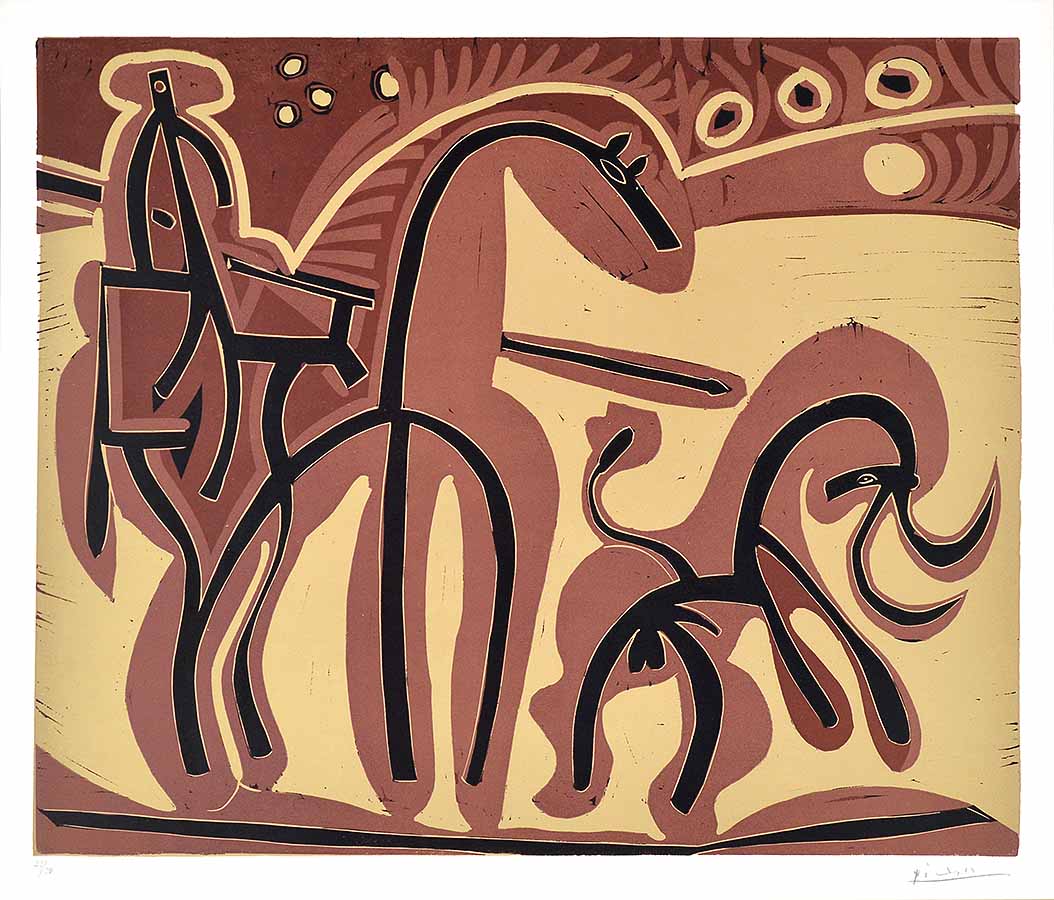This highly stylized artwork depicts a dynamic scene featuring a horse with a rider holding a spear, engaged in the chase of a male bovine, which could be a cow or a buffalo. The composition showcases a vivid palette of burnt orange and sienna, with the figures outlined in black against a creamy-colored background. The artwork appears to be aged, reminiscent of ancient engravings or illustrations one might find on an old urn from earlier historical periods. The rider is depicted seated on what appears to be a saddle, emphasizing the realistic elements melded with the stylized nature of the piece. Notably, the male bovine is clearly identifiable by its visible genitalia, adding an additional layer of detail to this evocative portrayal.